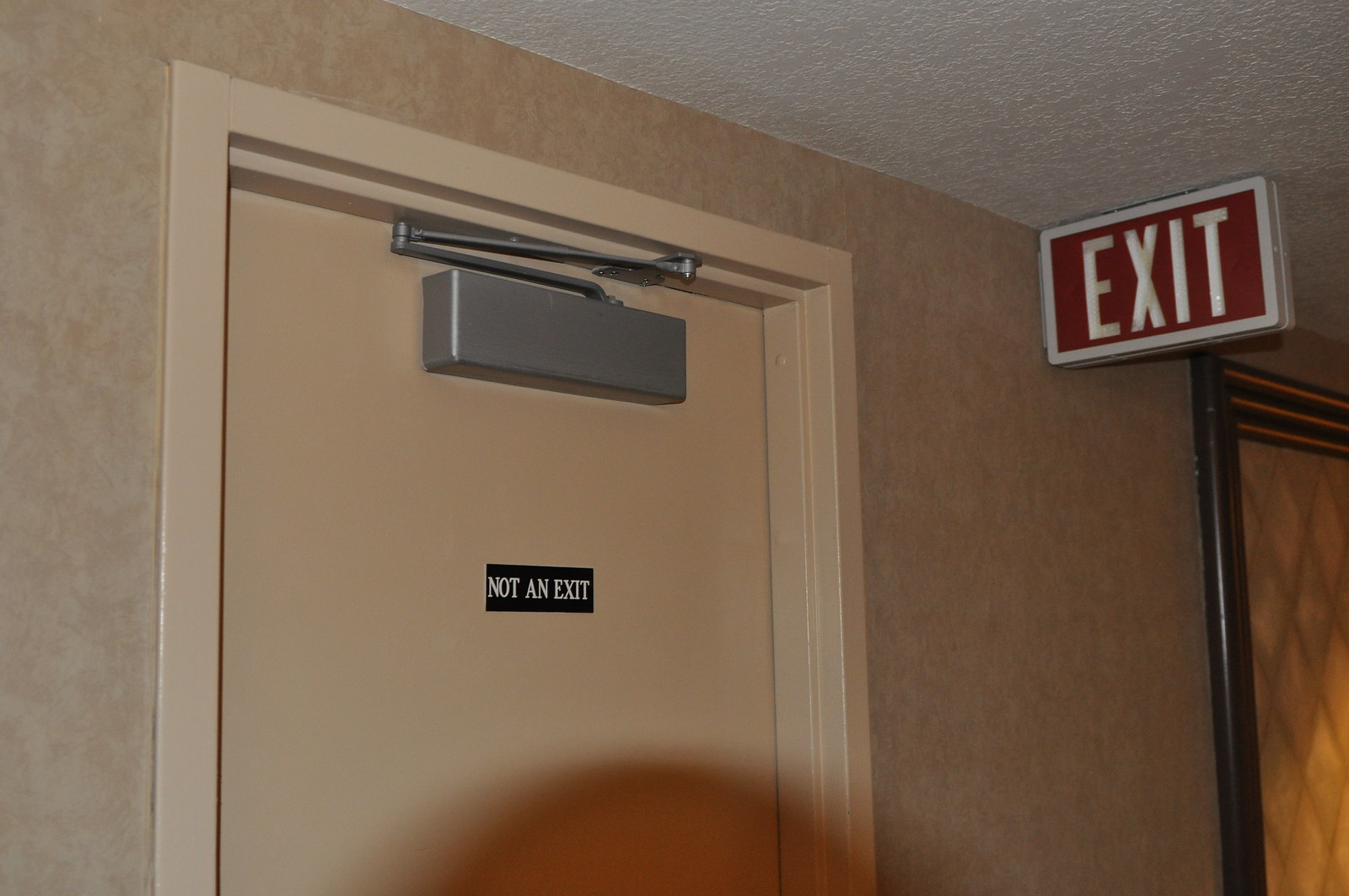The image depicts the interior of a commercial hallway characterized by beige textured walls and a white, popcorn-style ceiling. Central to the scene is a tan door equipped with a square-shaped, silver hydraulic hinge at the top. Contradictorily, despite the vibrant, red and white exit sign positioned near the ceiling just above the door, a small black plaque with white lettering firmly states "NOT AN EXIT." In the top right corner of the photo, the exit sign is clearly visible, underscoring the contradiction. Adjacent to and beneath the exit sign on the opposite side, a dark, possibly metal object is partially visible. The hallway also features an open doorway with black trim, suggesting another potential exit, although it remains unclear from the photo if it includes a door. A faint shadow, possibly of the photographer, extends across the door, adding to the complexity of the scene.